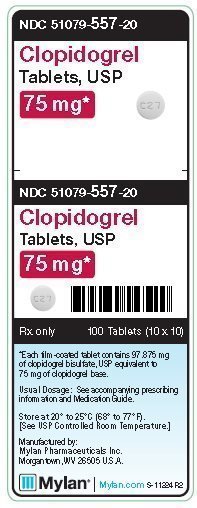The image displays a monochromatic medication label for Clopidogrel Tablets. The National Drug Code (NDC) labeled "51079-557-20" is prominently featured. The tablet, available in a 75-milligram dosage, is depicted beside the text with an engraving of "C27". This small, round, white pill is shown next to a black and white barcode. Below the barcode, it specifies that the medication is for "RX only," indicating that it is prescription-only. The packaging contains "100 tablets, divided into 10 groups of 10."

A section highlighted in light blue details the composition, stating, "Each slim-coated tablet contains 97.875 milligrams of Clopidogrel bisulfate USP, equivalent to 75 milligrams of Clopidogrel base." The usual dosage and further instructions reference the accompanying prescribing information and medication guide. Storage recommendations are provided, indicating the medication should be kept at a controlled room temperature of 20 to 25 degrees Celsius (68 to 77 degrees Fahrenheit), as per USP guidelines.

The label notes that the tablets are manufactured by Mylan Pharmaceuticals, Inc., based in Morgantown, West Virginia, USA. The Mylan logo and brand name are displayed at the bottom, along with the website "Mylan.com" in blue text, presumably clickable in a digital format. The document identifier "S-11224R2" appears in black at the bottom, and there is no additional information provided.